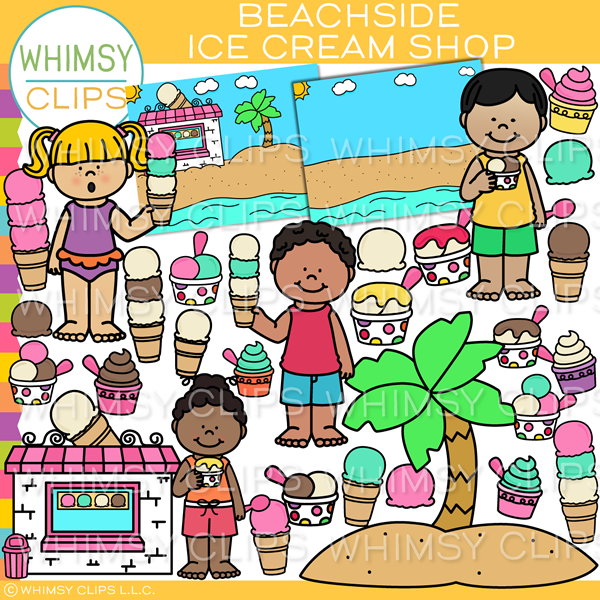This is a whimsical, computerized illustration titled "Beachside Ice Cream Shop" featuring four cheerful children enjoying their ice cream. The vivid scene displays the Whimsy Clips LLC copyright logo in the lower right corner, with the Whimsy Clips name superimposed over the entire image and its logo prominently positioned in the upper left corner. The lively beach setting showcases a variety of ice cream imagery scattered about, including cones with single, double, and triple scoops, as well as cups with different flavors.

At the forefront, a blonde girl in a purple bathing suit holds a tall triple-scoop cone, her hair gleaming in the beachside sun. Beside her, a boy in a green shirt and green shorts clutches a cup of ice cream. In the center, a barefoot boy sporting a red shirt and blue shorts proudly shows off his triple-scoop cone. Completing the group, a little girl with pink shorts and an orange top contentedly enjoys her cup of ice cream. The background is rich with details, including white ice cream stalls with pink roofs and a cheerful palm tree, further enhancing the playful, summer vibe of the scene.